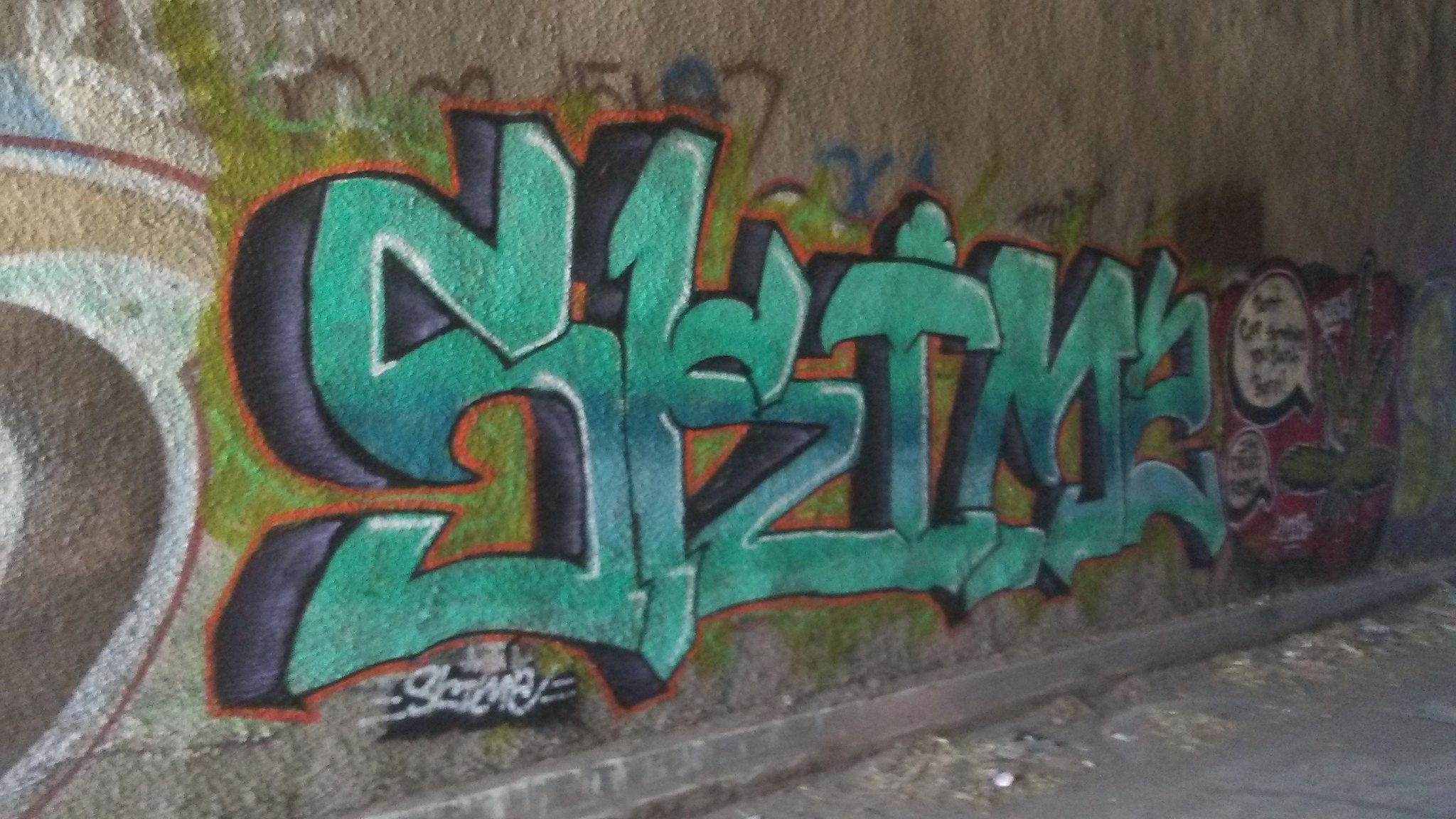This photograph captures a vibrant graffiti mural on a concrete wall, seemingly part of an urban underpass. The centerpiece of the mural prominently features the word "SLIME" in eye-catching, green spray-painted letters with a 3D drop shadow effect. The background of the wall appears gray, peppered with a multitude of graffiti pieces displaying a riot of colors. To the right of the central mural, another graffiti tag in turquoise block lettering, possibly reading "SKZTMZ," stands out. This piece is accentuated with a black shade and outlined in reddish-orange, signed by the artist in white letters at the bottom. Surrounding these tags are additional intricate designs, including a speech bubble and a red and white blob, adding complexity to the textured backdrop. The bottom right-hand corner of the image reveals a dirty sidewalk, grounding the scene in an outdoor, gritty urban environment.